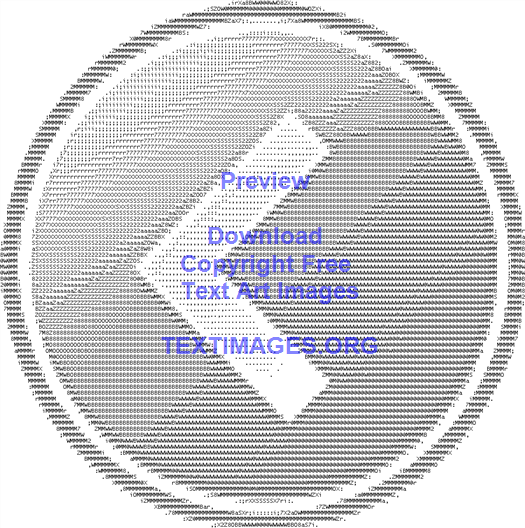The image showcases intricate ASCII art, featuring a circular design that resembles a 3D button. The exterior of this circular graphic is outlined with a dark border, followed by a concentric white border. Within the center, another smaller circle exhibits a gradient shading effect, transitioning from lighter tones at the top left to darker tones at the bottom right. At the very center of the inner circle, there is a white chevron symbol pointing to the left. The entire composition utilizes various printed characters to achieve detailed shading and depth. Overlaying the graphic, in blue font, is the text: "Preview. Download copyright free text art images at T-E-X-T-I-M-A-G-E-S dot O-R-G," adding a layer of informational content without detracting from the visual intricacy of the ASCII art.